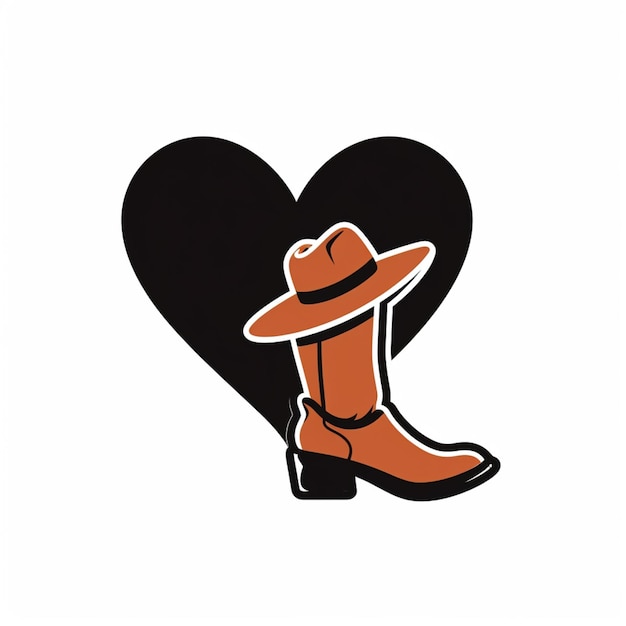The image is a digitally generated drawing, possibly resembling a logo or sticker. It features a centered black heart against a white background. Positioned in front of the heart is a single brown ankle-high boot, depicted from the side. The boot has a black heel, a black sole, and white lines near its boundary. On top of the boot rests a brown hat adorned with a black and white headband, tilted diagonally with the brim angling low to the left and high to the right. The overall composition is minimalistic, with no additional elements in the image.